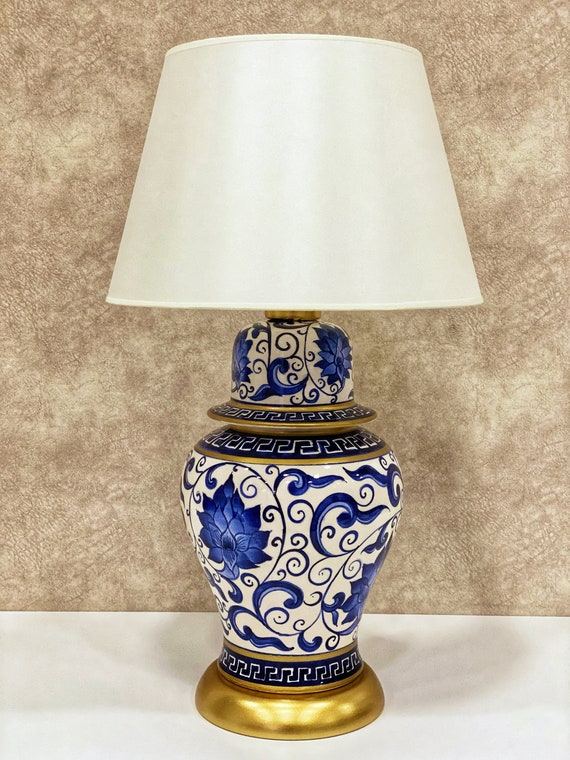This photograph captures a white lamp with a traditional white, angled lampshade, positioned on a pristine white table. The backdrop is a textured cream and tan wallpaper that lends an elegant contrast to the lamp's features. The base of the lamp is ornate, primarily white with intricate blue floral designs reminiscent of delicate china patterns. The blue design features elaborate swirls, curlicues, and a prominent blue lotus flower on the left side. Accentuating its sophisticated appearance, the bottom part of the lamp base is finished in a reflective gold paint, and additional gold bands adorn the top portion, enhancing its ornamental look. The lampshade itself appears smooth and crisp, reflecting a soft sheen that complements the meticulous artistry of the base, creating a refined and stylish composition.